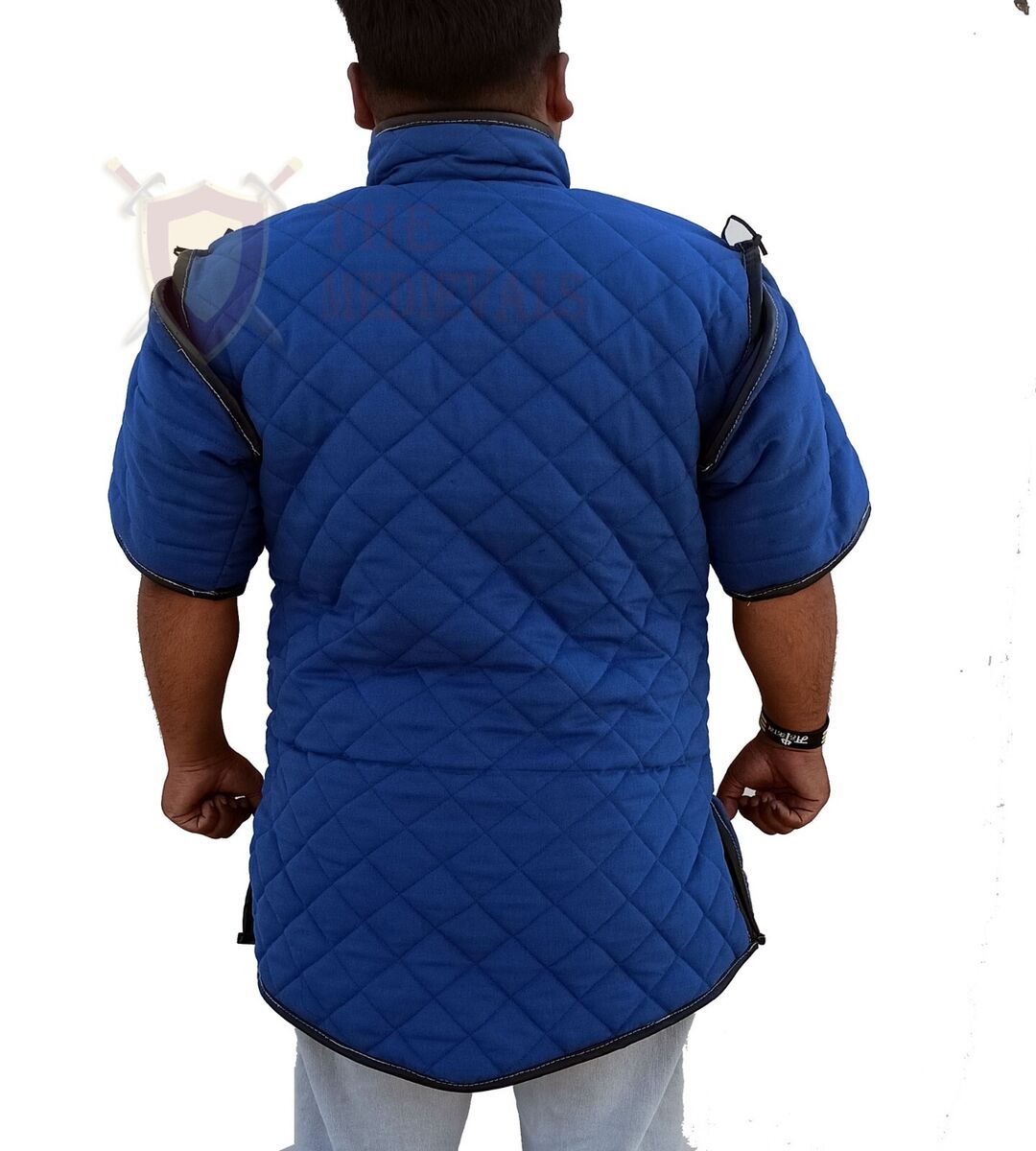The photograph features the back view of a dark-complexioned male with short-cut black hair. He is dressed in a quilted, short-sleeve jacket that is dark purple or possibly dark blue, marked by a distinctive diamond pattern. The jacket includes detachable sleeves with zippers and a collar that mirrors the hem of the jacket. Along the upper arms of the jacket, there is a thick black tubing-like strap. Additionally, there is a logo on the jacket—a transparent shield with two swords crossed behind it. The man is also wearing gray sweatpants or potentially loose denim pants. On his right wrist, he adorns a black bracelet with noticeable large white lettering. His hands are clenched into fists, not resting or relaxed.